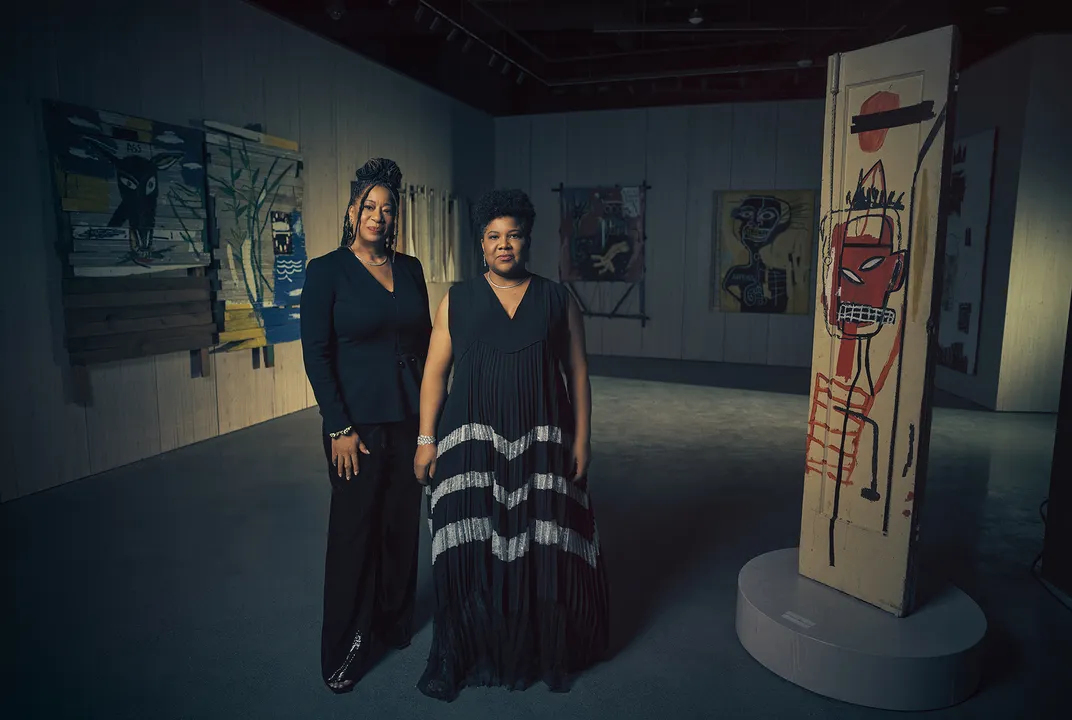The image depicts two women, both with dark brown or black hair and brown skin, standing in a dimly lit art gallery. The woman on the right wears a floor-length, sleeveless black dress with a v-neckline and three horizontal white patterns just below the hips, giving the dress a flowing appearance. The woman on the left is dressed in a dark suit with a jacket and a skirt. The gallery setting features ethnic artwork in bold primary colors—reds, blues, yellows, and blacks—displayed on various non-traditional materials. The lighting is dramatic, casting a yellow and almost blue tint, suggesting the gallery is closed with focused lighting illuminating the women while the rest of the space remains in shadow. The artwork behind them is primal and vibrant, adding a dynamic and cultural backdrop to the scene. The overall composition suggests a professional photographic setting, possibly meant for promotional purposes related to the art exhibition or the artists themselves.